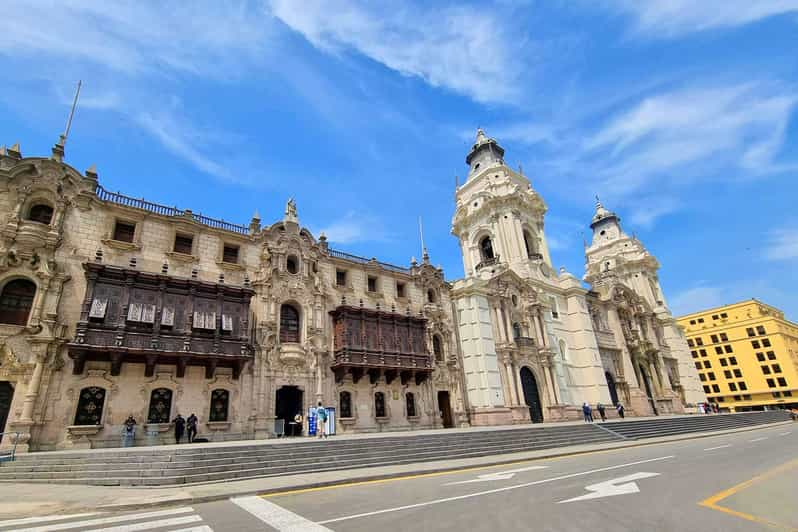This image, taken from across the street with a slightly upward angle, depicts a grand, ornate building that occupies an entire city block. The structure is reminiscent of Baroque architecture, suggesting it might be a significant landmark such as a government building, palace, library, or museum. The facade is primarily constructed from light-colored beige stone, worn and aged, with intricate designs featuring columns and arches spaced at intervals. The building exhibits architectural variations, including towers or spires that rise from the central structure, contributing to its elaborate aesthetic.

On the right-hand side, there's a visually distinct section made of beige concrete, appearing closely attached but possibly a separate structure. This section includes an archway supported by detailed columns, adding to the complexity of the architecture. The street in front of the building, marked by a double left-hand turn lane, leads up to five steps ascending to a spacious, elevated plaza parallel to the road. The photograph also captures a handful of pedestrians on the sidewalk, providing a sense of scale to the immense building. Behind this majestic structure, a modern five-story yellow building with rectangular windows contrasts sharply with its historical counterpart, all set against a light blue sky with wispy clouds.